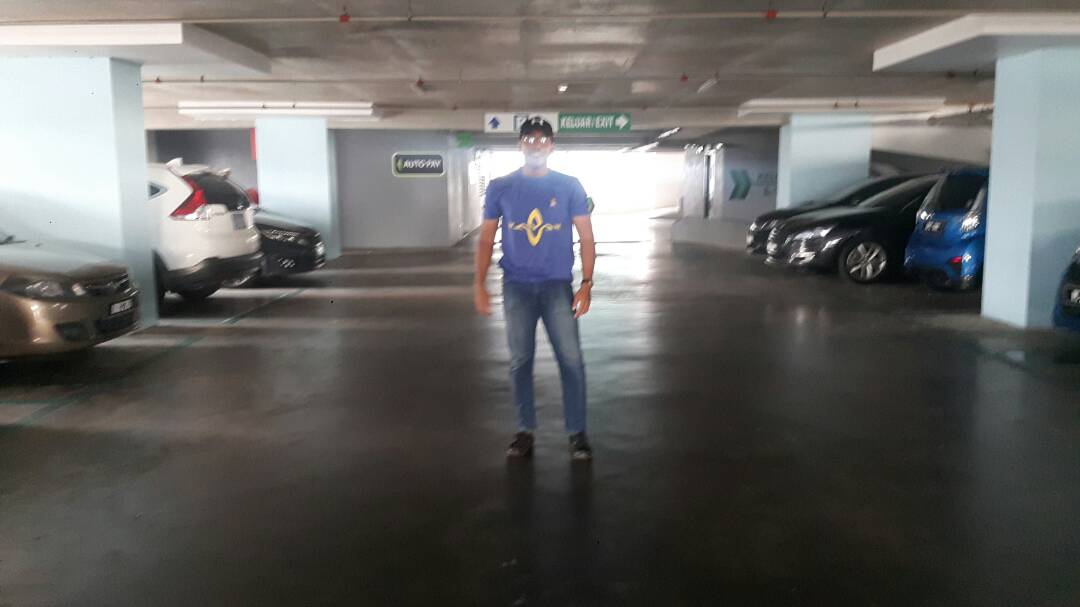In this detailed photograph of an underground parking garage, a man stands centrally in the middle of the drive lane, facing the camera with his arms hanging straight down at his sides. He is smiling slightly as his picture is taken. The garage's gray concrete floor stretches beneath his feet, while cars occupy every visible parking space around him. 

The man is wearing a short-sleeved blue shirt adorned with a distinctive yellow oval logo featuring a wave-like design. Underneath, he has a blue t-shirt and blue jeans, complemented by black shoes. He sports a black baseball cap, emblazoned with a white logo, and a pair of glasses. Additionally, he wears a wristwatch on his left arm. 

Behind him, a significant light source floods in through the exit, obscuring some details of his face. Clear signage, including an "Exit" sign with an arrow pointing to the right near his head and an "Auto Pay" sign pointing left, is visible on the walls. The walls boast a blue color with white outlining borders above them, and support pillars punctuate the space.

Vehicles seen include the front of a brown car on the right, the back of a white SUV farther to the right, and an array of other cars spread across visible parking spaces, notably two black cars and the back of a blue SUV. The ceiling matches the gray tone of the floor, enhancing the utilitarian ambiance of the garage.